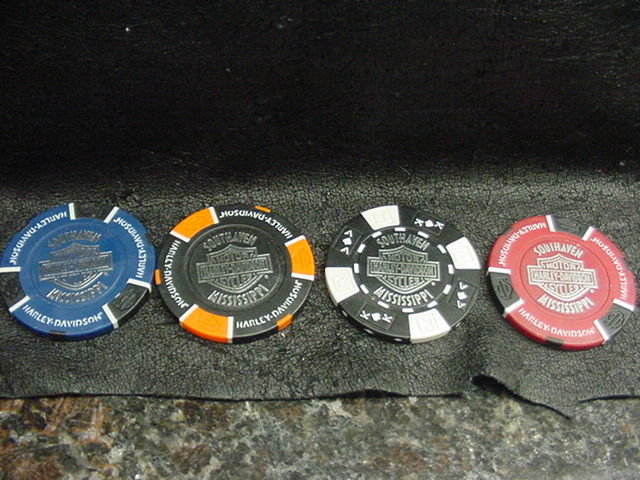This detailed photograph showcases a set of four poker chips or coin-like badges, aligned horizontally across the image, with the leftmost just slightly cropped by the edge. They sit atop a piece of black textured fabric, which lies on a stone countertop. The badges share a common design, each featuring the Harley-Davidson logo prominently in the center. The text "South Haven" arches above the logo, while "Mississippi" curves below it. The outer rim of each badge contains additional text, although it is largely illegible.

Starting from the left, the first badge is predominantly blue with three black rectangles bordered by white stripes around its edge. The next badge combines black and orange, with black rectangles bordered in orange and white. The third badge is mainly black, distinguished by four white rectangles on the border, with interspersed black sections depicting a playing card design—letter 'K' in the top left and bottom right corners, and a club symbol in the center. The final badge on the far right is red, featuring black rectangles with white stripes along the border, and also includes "Harley-Davidson" text in red on its rim.